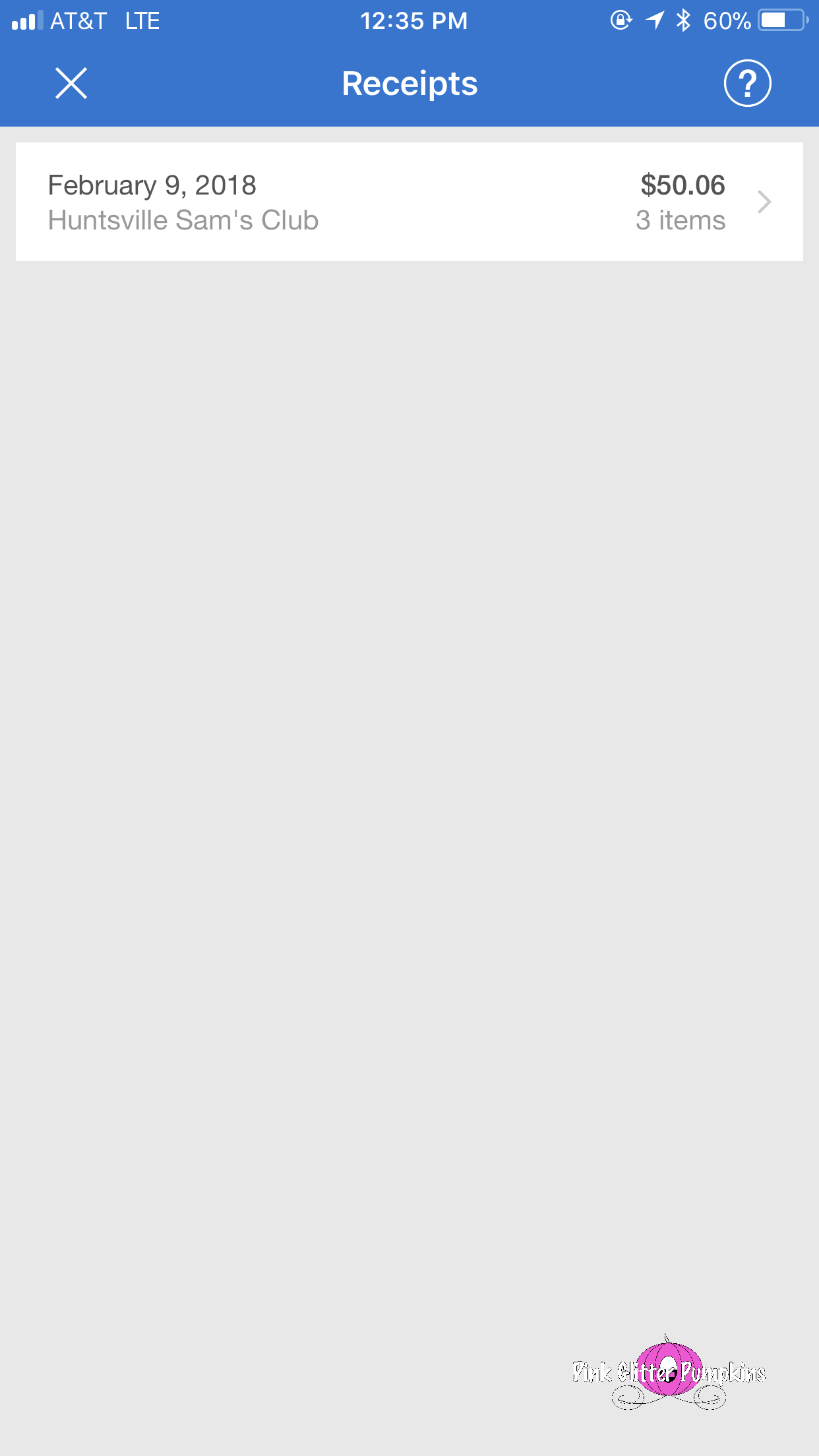Screenshot of a mobile receipts page, displaying a detailed transaction record. At the top of the image, there is a prominent blue bar with the word "Receipts" centered in white text. To the left of this text, there is an 'X' icon, while a question mark icon enclosed within a circle is situated on the right side. Below this blue bar, the interface includes a gray section. 

Within this gray section, there is a highlighted white box containing the receipt details. The receipt is dated February 9, 2018, with the store listed as "Huntsville Sam's Club." The right side of the white box indicates that the total amount of the transaction is $50.06 and mentions that three items were purchased. A forward arrow icon is located to the right of this text, suggesting that further details or actions can be accessed.

At the bottom of the screen, a distinctive logo features the text "Pink Glitter Pumpkin" accompanied by a pink pumpkin illustration.

Additionally, the device’s clock shows the current time as 12:35 p.m., positioned above the blue bar labeled "Receipts."